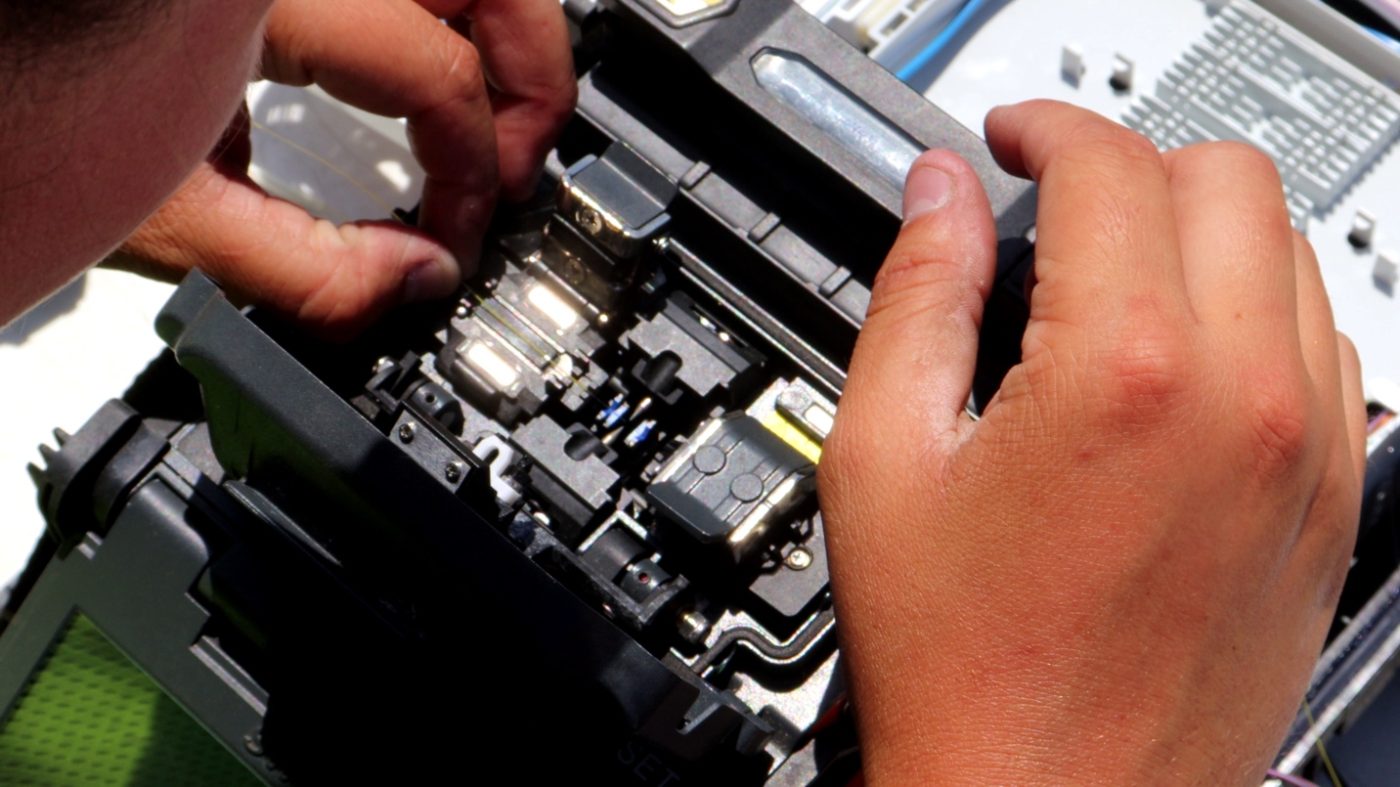In this image, we observe a person carefully working on an electronic device or some mechanical project. From a bird's-eye view, the person's face is partially visible in the top left corner, showing their cheek and a bit of their hair. Both of the individual's hands are engaged in the task, with the right hand being more prominently seen. They appear to be leaning over a black box with a plastic encasing, which contains a variety of metal components and shiny silver elements indicative of circuitry.

The device they're working on seems to be part of a larger machine, given the presence of a white piece of metal with slots and grooves located at the top right corner of the image. Running along the center portion of the photo, a blue wire can be seen. Inside the black box, there are blue fuses, wires, and screws, as well as white lights and silver ridges.

In the background, hints of other electronic devices are visible, including what looks like a computer board or similar equipment. On the bottom left, a green, possibly bumpy cloth or table surface is present, supporting the workspace. This detailed and realistic photograph captures a precise moment of meticulous craftsmanship and technical engagement.